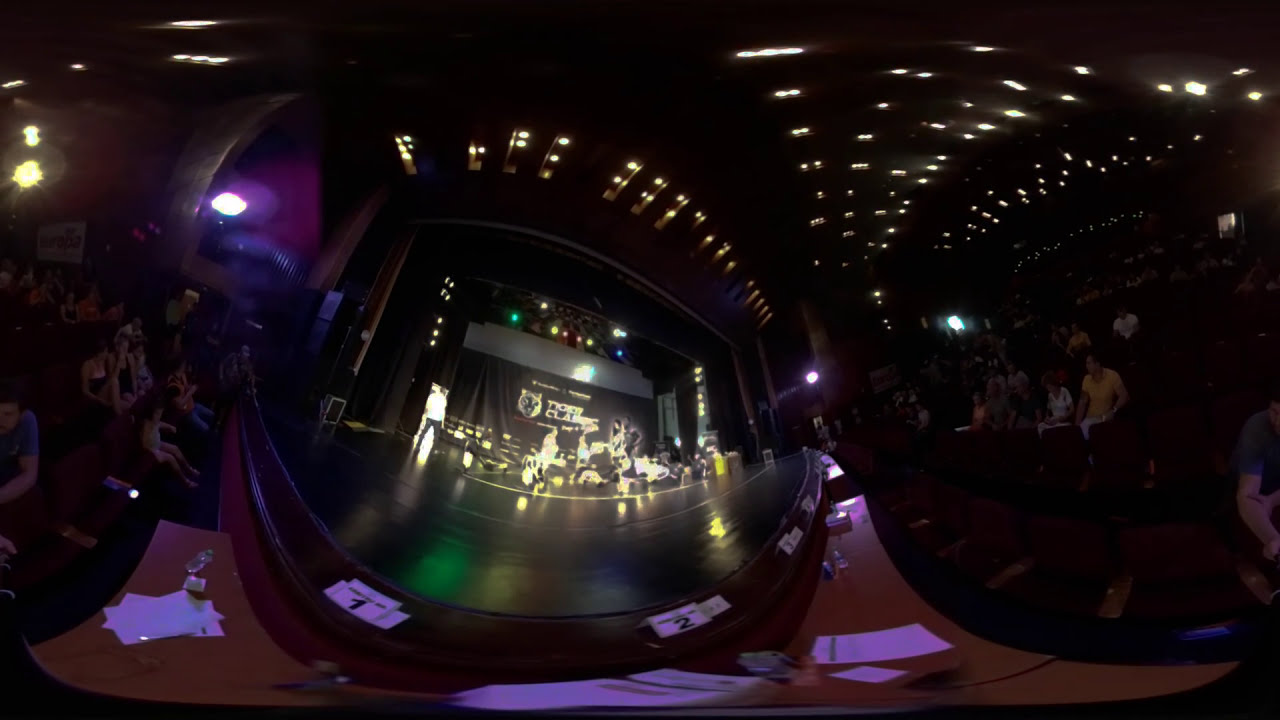The image captures a darkly lit theatre featuring a staged performance, likely a dance group, surrounded by an attentive audience. The central focus is on the stage, where approximately ten performers are illuminated by spotlights from the ceiling, their movements suggesting a dance routine. The image appears to be edited with a fishbowl effect, possibly through Photoshop or a specialized lens, giving the scene a distinctive circular distortion. On either side of the stage, around thirty audience members, predominantly Caucasian, are seated and watching intently. The theatre's ceiling is adorned with strands of white lights, creating a starry effect. In the background, a banner displaying the words "Tiger Glass" alongside an image of a tiger head is visible. Despite some visual ambiguities and glowing fluorescent colors, the performers are discernible. The purple hues and comprehensive 360 imaging add to the dynamic, somewhat surreal atmosphere of the photo.